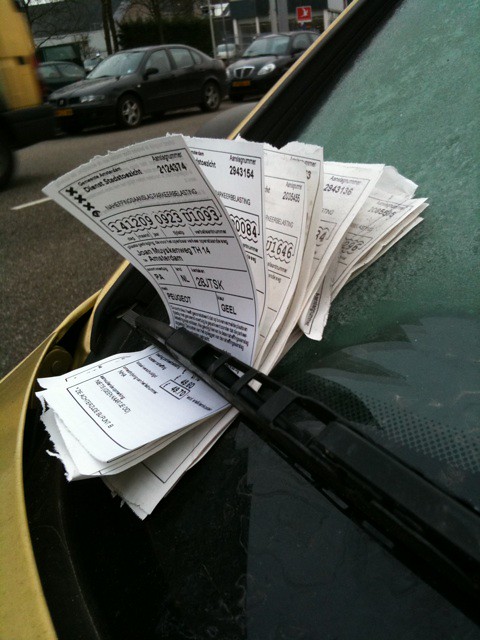The image captures a close-up of the front side of a car with a golden or yellow-green hue, parked in what appears to be a cold and rainy environment. The windshield wiper is clearly visible and holds a thick stack of white papers, presumably parking tickets or fines, each marked with various numbers and some text that’s not in English. The topmost ticket displays a total amount of $49.70. The windshield itself is frosted, indicating chilly weather. In the top left corner, there's visible traffic on a road, with a body of water, a hill, and a few trees in the background. A red and white sign, along with a striped white line going down the center of the road, can also be seen. This detailed composition suggests the car has been unattended for a prolonged period, accumulating multiple fines.